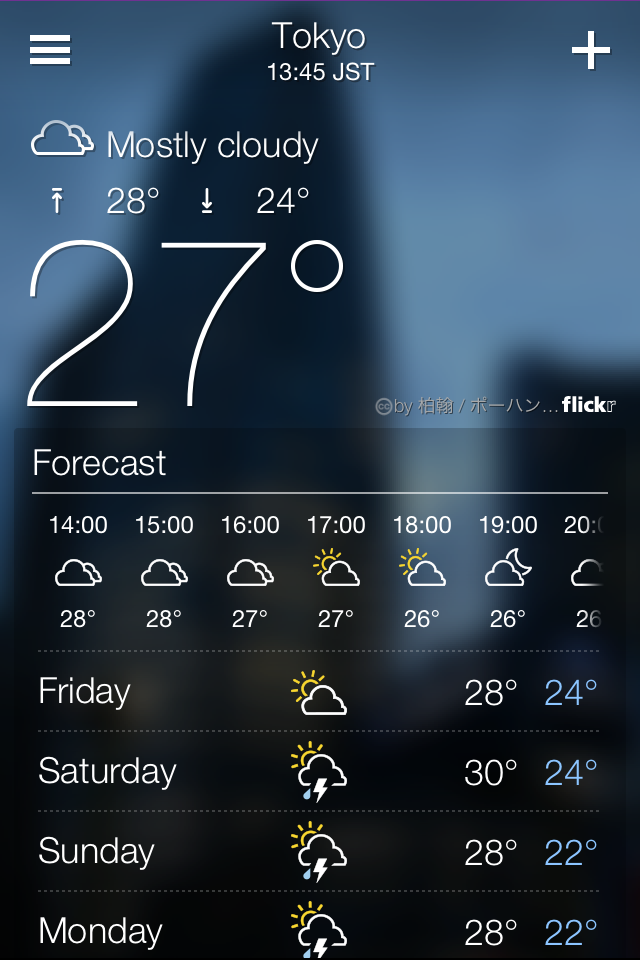A typical weather application screen displayed on a cell phone for the city of Tokyo. The background is a dark blue, almost black, with the text "Tokyo" at the top, specifying the location. The current time is indicated as 13:45 JST (Japanese Standard Time). On the left side, there are three horizontal bars symbolizing a menu, and on the right, there's a plus sign, likely for additional options.

The forecast prominently shows that the weather is mostly cloudy, represented with small cloud icons. The temperature readings include a high of 28°C (indicated with an upward arrow) and a low of 24°C (indicated with a downward arrow). The current temperature is displayed in large numbers as 27°C. Adjacent to the temperature, some text in Japanese is accompanied by the word "flick".

Below this, there is an hourly forecast from 14:00 to 20:00, showing fluctuating cloud coverage with occasional partial sunlight, alongside their respective temperatures. Additionally, there are options to view extended forecasts for the coming days (Friday, Saturday, Sunday, Monday), each selectable for an hourly weather breakdown.